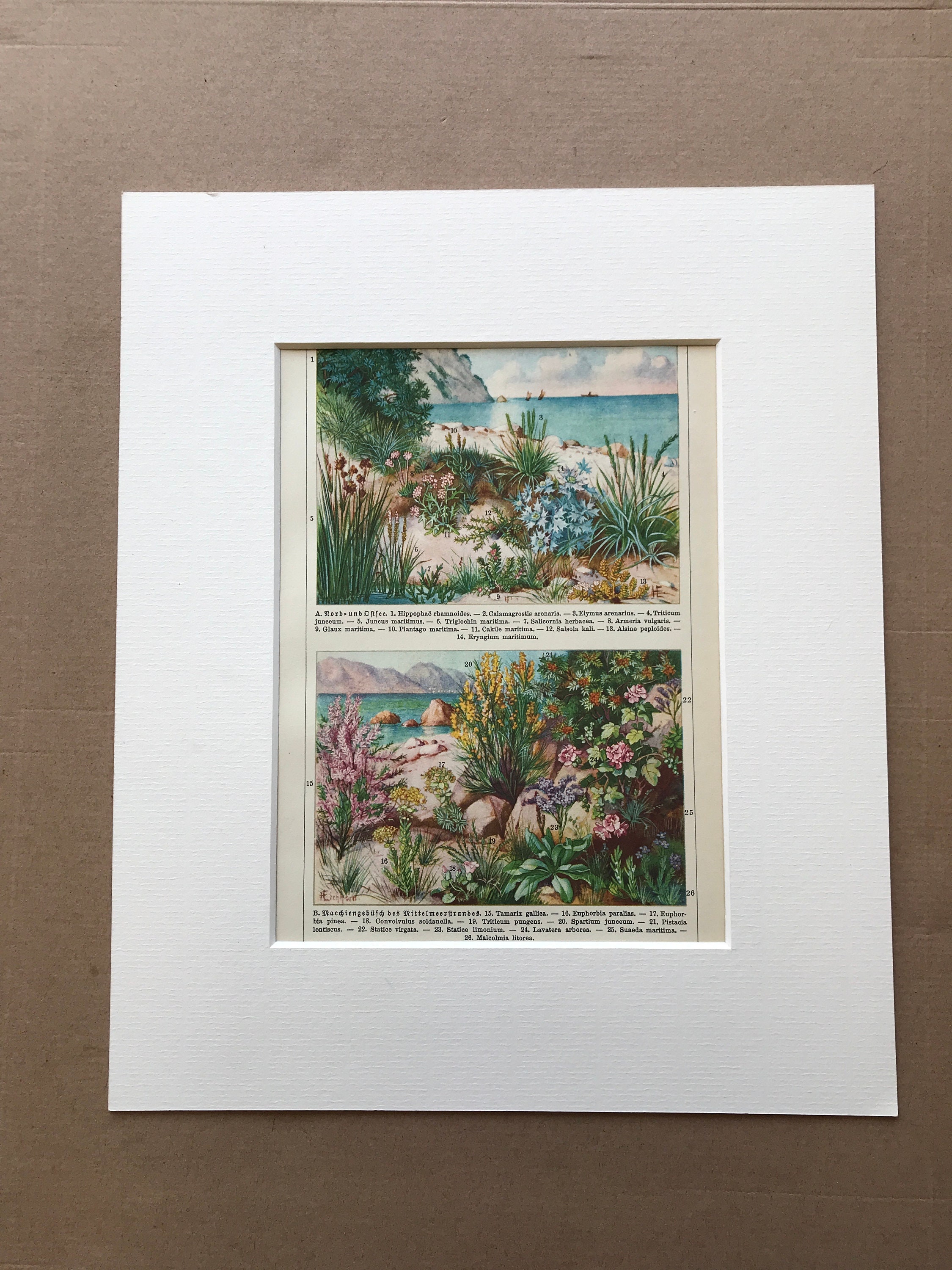This photograph captures a matted display of two illustrated, detailed watercolor scenes, set against a brown background which could be a wall or table. Enclosed within a thick white matte, the artwork lacks a frame. Both illustrations, painted directly on the same page, depict lush plant life at a beach shoreline. The top image presents a scenic view of mountains, clouds, and ocean waves, with various flora in shades of green, blue, and red. The lower illustration features a more concentrated collection of flowers in hues of yellow, pink, purple, and red, interspersed between rocks and set against a mountainous backdrop. Both images are accompanied by small, illegible labels beneath them, presumed to identify the depicted plants. The entire presentation conveys a rich, natural environment teeming with vibrant vegetation and serene coastal elements.